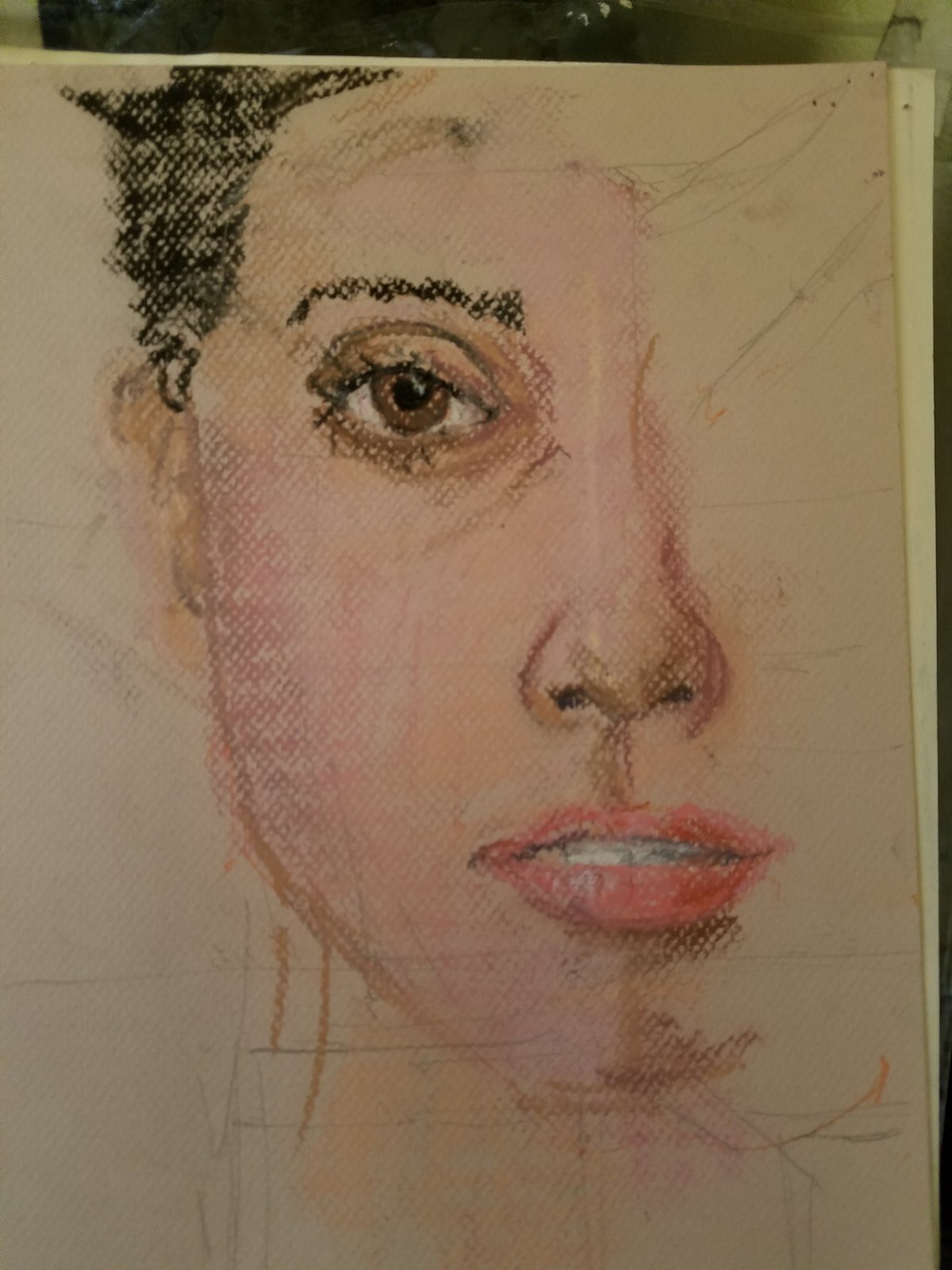This vertical image showcases a pastel drawing of a partially obscured female face, executed on a textured board. The artwork features the left side of the face in detail, with the full lips depicted in a frontal view, revealing the right half of the lips. The lips, colored a vibrant red, are parted slightly to display some of the teeth. The depicted eye is a deep brown, underlined by a dark, narrow eyebrow. The subject appears to be a Caucasian woman, suggested by her flesh tones and the portrayal of her short, black hair. The artist has skillfully used flesh tones and shades of brown to create realistic shading, giving the face a three-dimensional appearance. Overall, the proportions are harmonious, and the drawing is rendered with notable skill and detail.